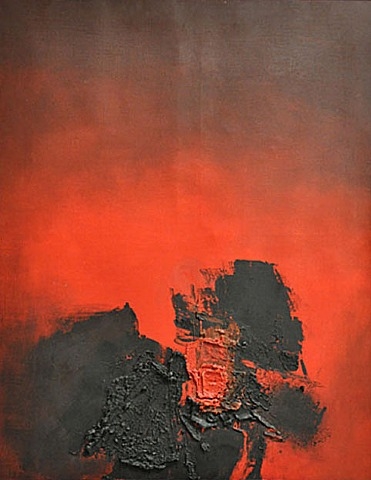This image is an abstract modern painting featuring a prominent gradient backdrop and bold brushstrokes. The top of the canvas starts with a deep brown hue that transitions smoothly into a vibrant crimson red, evoking the intensity of a fiery sky. The red portion is centrally located, especially towards the lower middle section, and is covered by a soft, smoky filter that adds depth to the upper part of the painting.

Dominating the bottom left and extending slightly to the right is a large, textured black smudge, reminiscent of thick tar or oil. This area has varying textures: the left side appears more faded and matte, while the right side looks more clumped and shiny, as if the paint was applied heavily. The black brushstrokes are aggressive and thick, creating a stark contrast against the vibrant red background. There are some indentations within the black paint, adding an extra layer of complexity to the texture. Overall, the painting's rough textures and bold colors create a dynamic and intense composition.